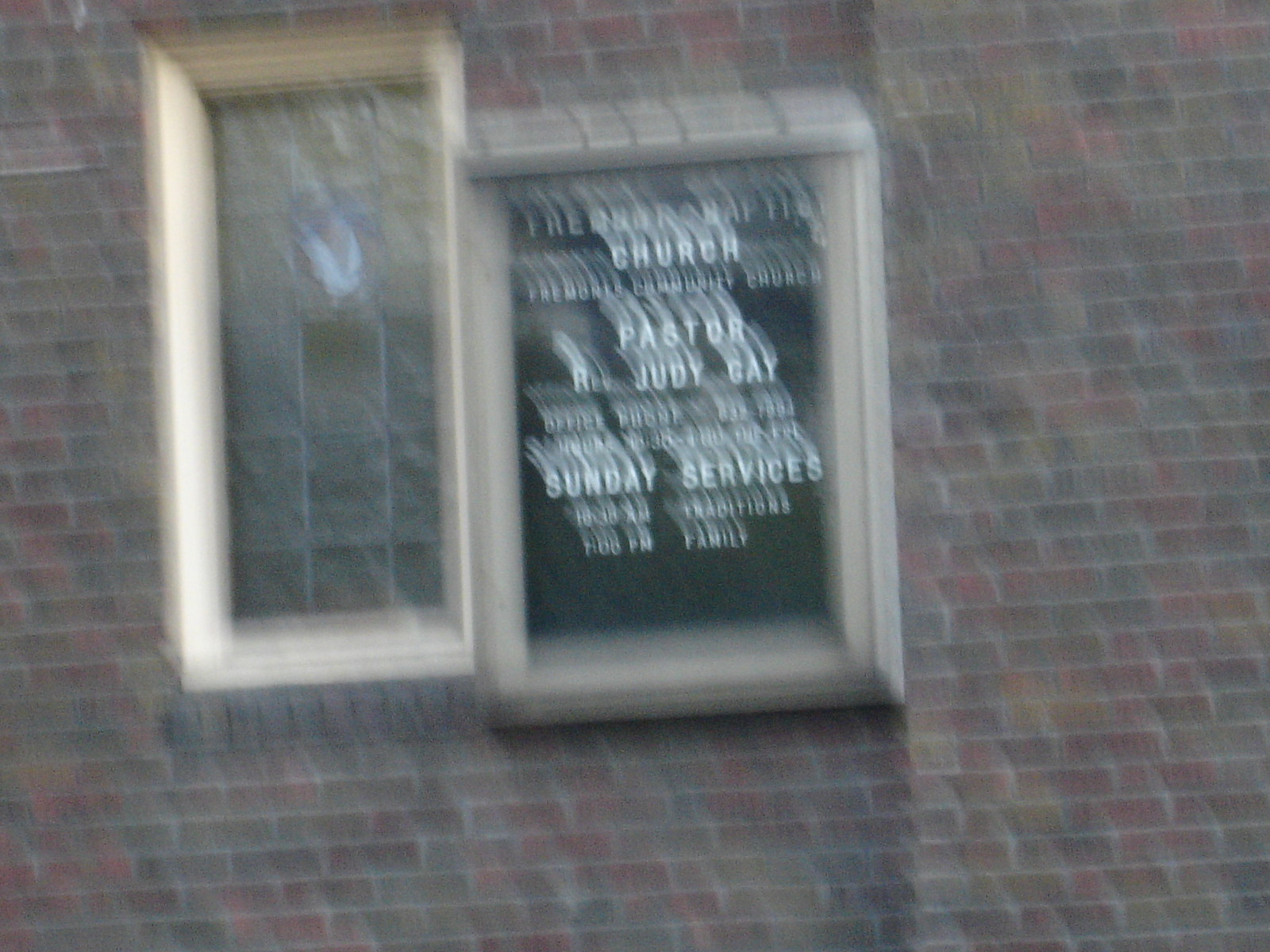An image of a brick building featuring three windows in total—one on the left side, and two on the right. Mounted on the building is a rectangular, wooden-trimmed sign with a black background, though it is somewhat blurry. The sign appears to read "The Free Church" or something similar. Below this, it indicates the pastor's name as Reverend Judy Gay. Additionally, the sign lists the church's service times, noting Sunday services at 10:30 a.m. and a family gathering at 7 p.m.